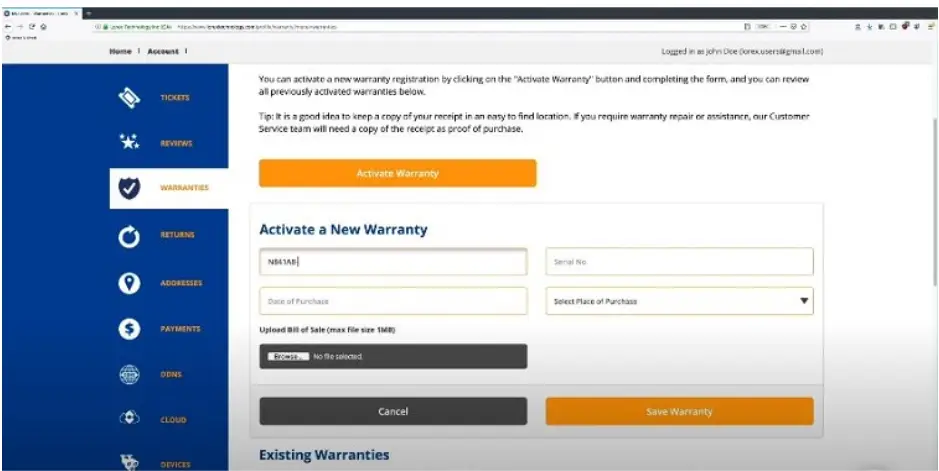Screenshot of a predominantly white webpage with a blue sidebar featuring various categories in gold text. The categories listed are Tickets, Reviews, Warranties, Returns, Addresses, Payments, DNS, Cloud, and Devices, each accompanied by a corresponding icon. The Warranties category is highlighted, indicating the current section, with a shield icon bearing a white checkmark. On the right side of the page, there's a form for activating a new warranty. An orange button labeled "Activate Warranty" is prominently displayed above four input fields for entering necessary information to complete the activation process.